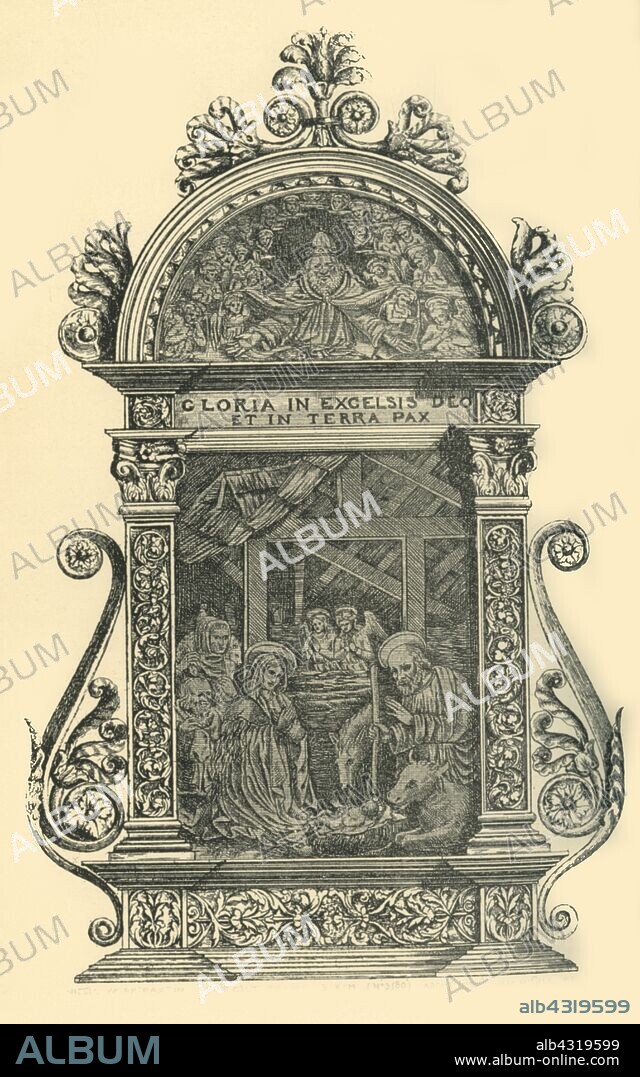The image is a hand-drawn depiction of an ornate stone shrine, structured like a cross-section revealing an intricate interior scene. The backdrop is a pink hue, repetitively watermarked with the word "album" diagonally. The sketch, likely representing a statue or similar artwork seen outside a church, portrays the nativity scene at its core. A banner reading "Gloria in Excelsis in Dio et in Terra Pax" arches above the scene. Surrounding the intricately carved nativity tableau are rich arrays of floral trims and elaborate inscriptions. Tall, decorative pillars flank the sides, supporting a rounded dome adorned with detailed carvings, giving a glimpse of its ornate design. At the upper interior arch, a depiction of God with outstretched arms is surrounded by angels. The artwork also includes shepherds, angels, animals, and other nativity elements. The lower right corner features the text "ALB4319599" and a URL "albumonline.com," while a black bar at the bottom left displays "ALBUM" in capital letters.